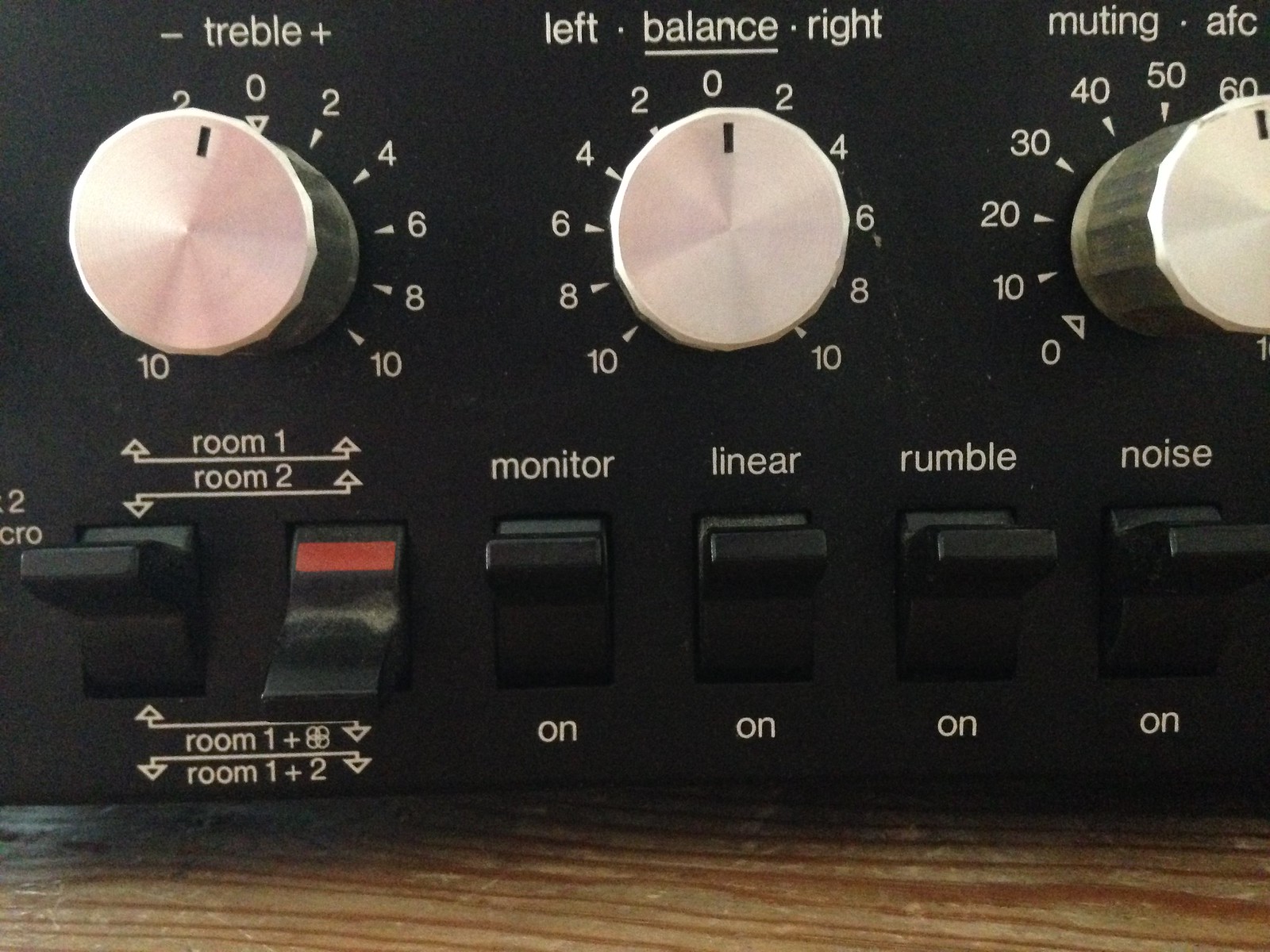This detailed close-up image showcases the front panel of a professional black stereo receiver, situated on a wood grain surface. The top section features three prominent silver knobs. The left knob, labeled "Treble," ranges from -10 to 10 with a black indicator line positioned slightly to the right of zero. The middle knob, labeled "Balance," ranges from left to right, marked from 0 to 10 in both directions, and is currently set at zero. The right knob is labeled "Muting" and includes an AFC dot; it spans from 0 to 60, with 50 approximately at mid-point.

Below these knobs, the panel includes several switches. To the left, two switches are labeled "Room 1" and "Room 2," designed for controlling different room settings. To the right, four on-off switches correspond to "Monitor," "Linear," "Rumble," and "Noise." Each of these switches displays "On" when engaged. Together, these controls and switches suggest a high degree of functionality for adjusting sound quality and distribution across different spaces.